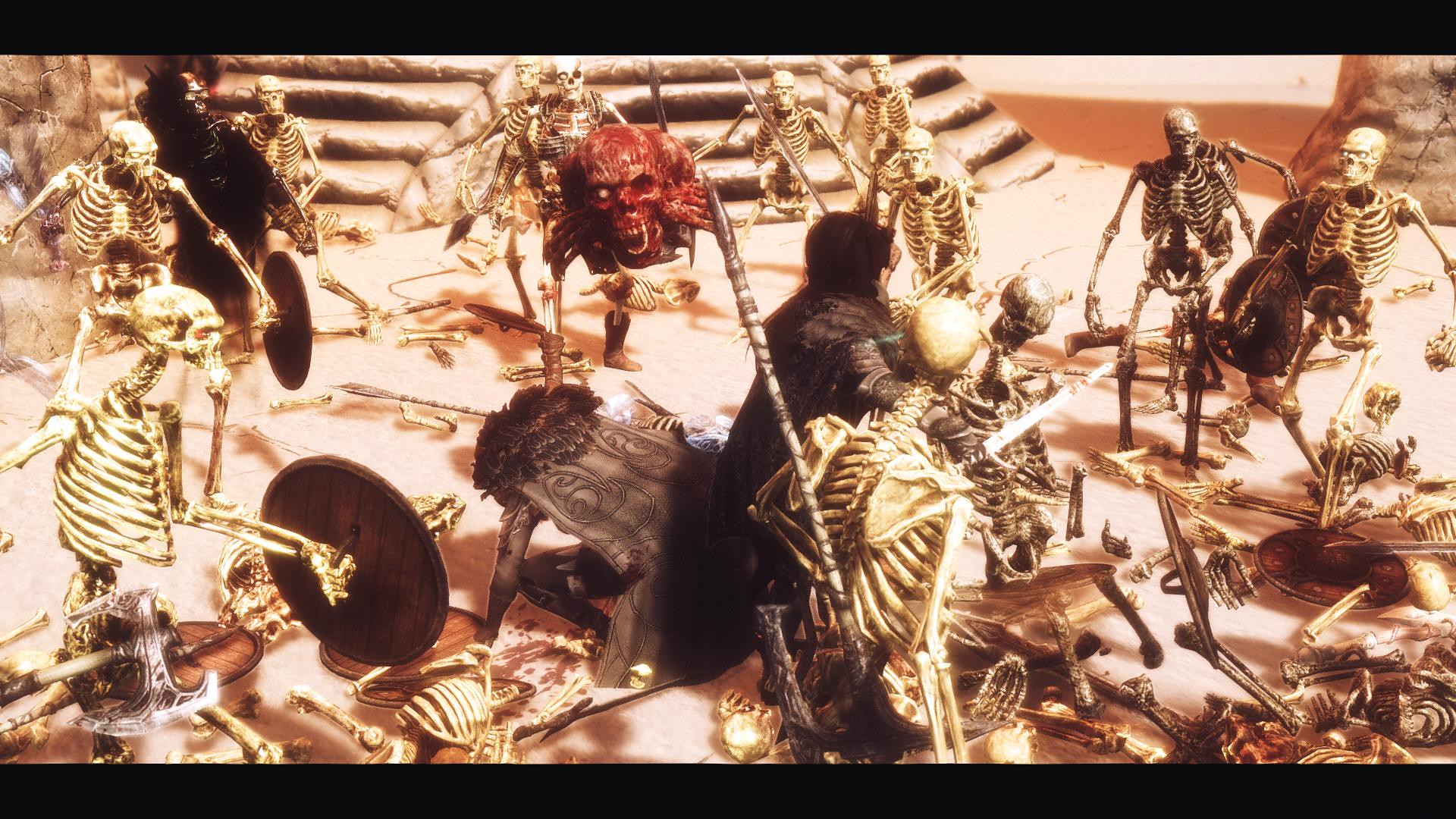The image depicts a detailed and dynamic scene featuring toy-sized skeleton models, engaged in combat. The majority of the skeletons are white or beige, with notable exceptions including a gold skeleton and a red skeleton-monster hybrid. A black skeleton also adds to the diversity in the display. The skeletons are equipped with shields, swords, and various other weapons, and are positioned in various states of battle, with some standing and others appearing broken or laying on the ground. One particularly striking element is a red skeleton head impaled by a sword, held aloft. All these figures are set against a pinkish backdrop, potentially indicating a display in a museum or a scene crafted for a movie. The setting is meticulously detailed, with a focus on the combat between these skeletal figures.